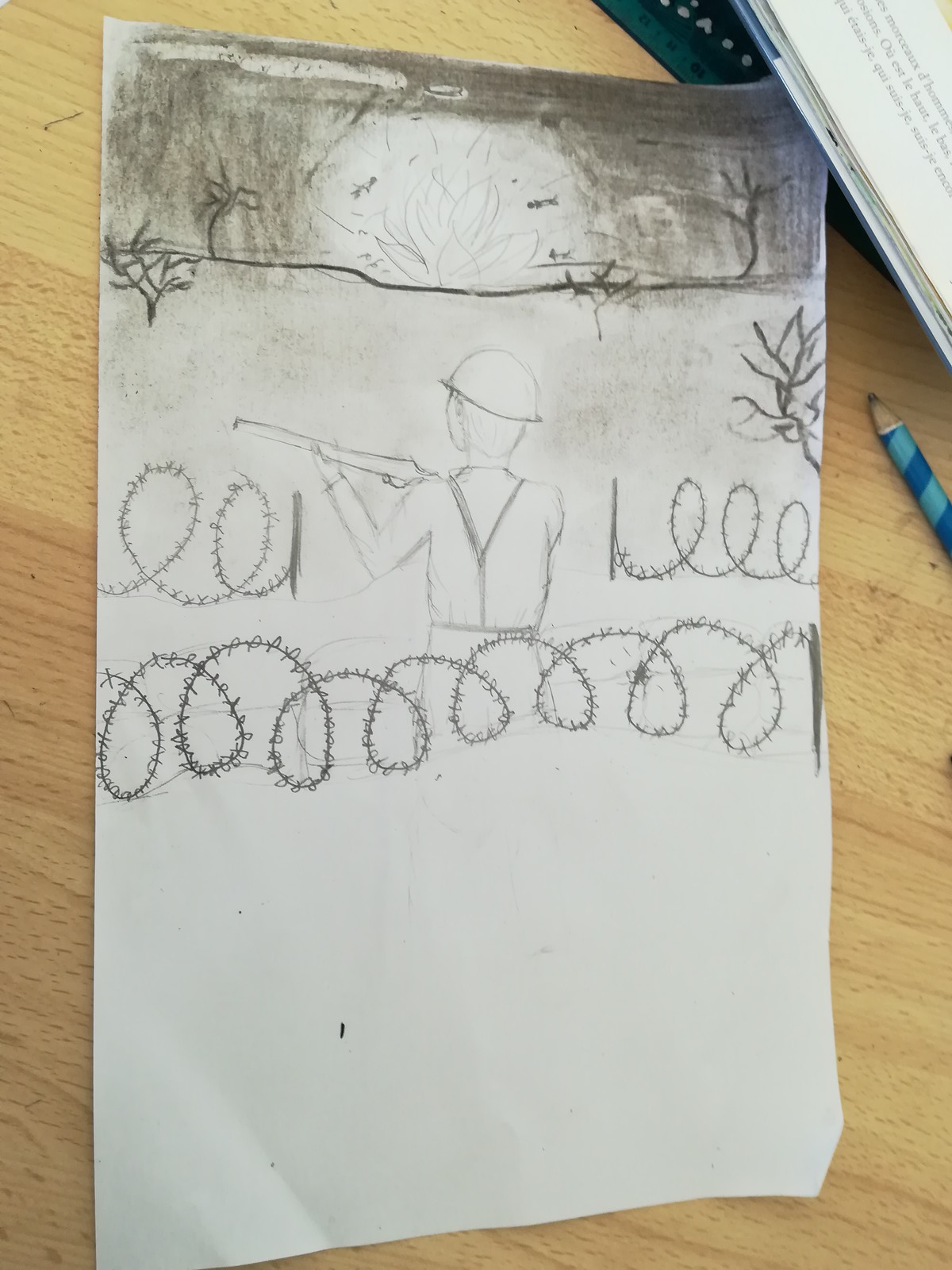The image depicts a close-up of a light beige wooden table or desk. On the right side of the frame lies a sharpened pencil with a light blue and dark blue spiral stripe pattern. Adjacent to it is a partially visible greenish ruler with indistinct markings. A rectangular piece of paper, the main focus of the image, showcases a pencil drawing. The drawing, which appears amateurish, captures the chaotic scene of a war zone. It features a soldier wearing a helmet, positioned amidst barbed wire coils and holding a gun. The background of the drawing is filled with dark, smoke-like smears, with hints of flames and several trees scattered across the scene. There's also a portion of an open book visible, with French text that includes "La Haute" in black.